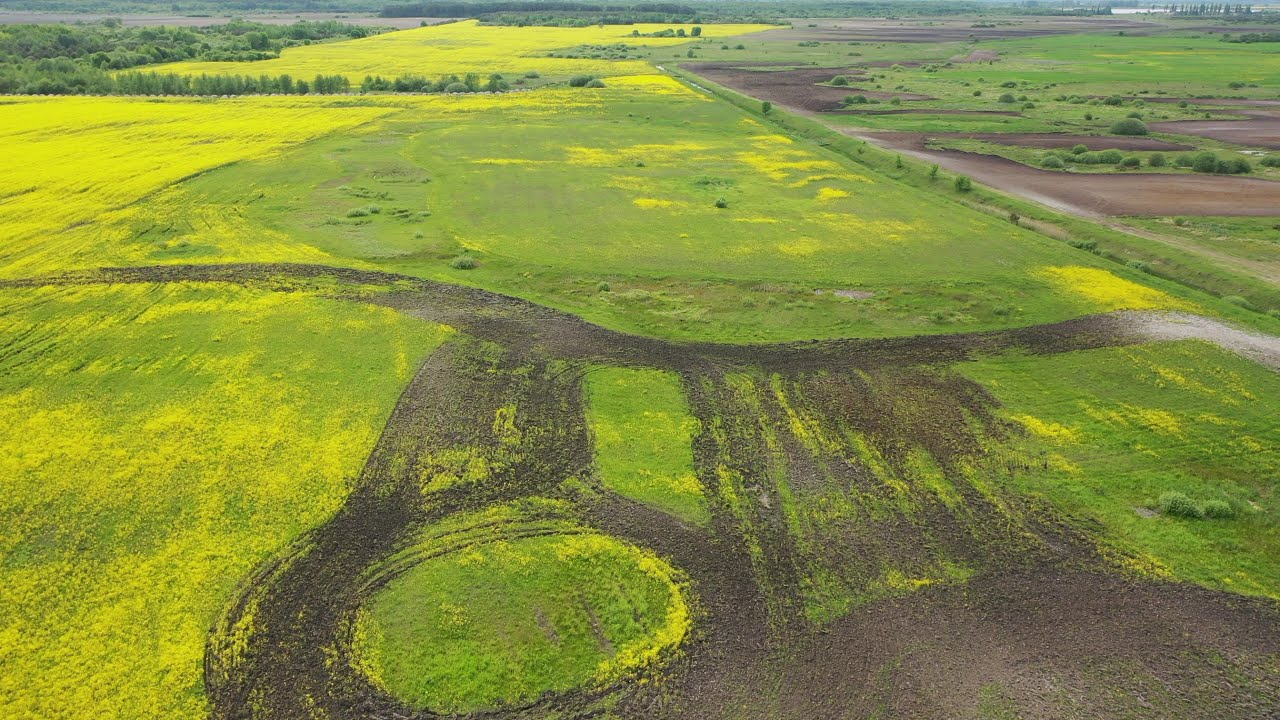This image is a high-angle aerial shot, likely taken from a drone, capturing a vast expanse of farmland. The majority of the landscape is a bright, vibrant green, interspersed with patches of yellow from wildflowers. The photo features a network of intersecting dirt roads and paths, with one prominent gravel road cutting across the bottom of the frame, noted for its dark brown hue with some areas appearing scarred.

Directly below, a circular pattern is evident in the grassland, hinting at activities like vehicles driving in circles, potentially for recreational purposes or as a result of farming equipment. This distinct circle adds an interesting texture to the scene. 

In the distance, this expansive grassland stretches off for miles, subtly segmented by rows of trees and additional fields. The left side of the image is dominated by the bright green field, while the right side, especially the upper right corner, shows a mix of darker greens from bushes and trees. There is also a waterway that can be seen running from the center-right toward the middle of the image, adding another layer of detail to the primarily flat terrain.

Overall, the landscape is a mix of greenery, dirt paths, and sporadically placed trees and bushes, showcasing a picturesque, meticulously structured farmland.